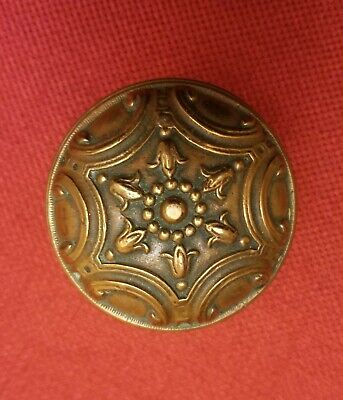The photograph depicts a large, ornate brass button or possibly an ancient artifact, centrally positioned against a textured red fabric, likely resembling a tablecloth with a visible grid pattern. This intricate round object features a symmetrical design: at its very center lies a singular circle, which is encircled by multiple smaller circles. Surrounding these is a hexagonal outline, with six tulip-like emblems extending outward. Additionally, six partially visible semi-circles can be seen curving inward towards the center along the outer edge. The detailed etchings and symmetrical patterns suggest this piece is both old and meticulously crafted.